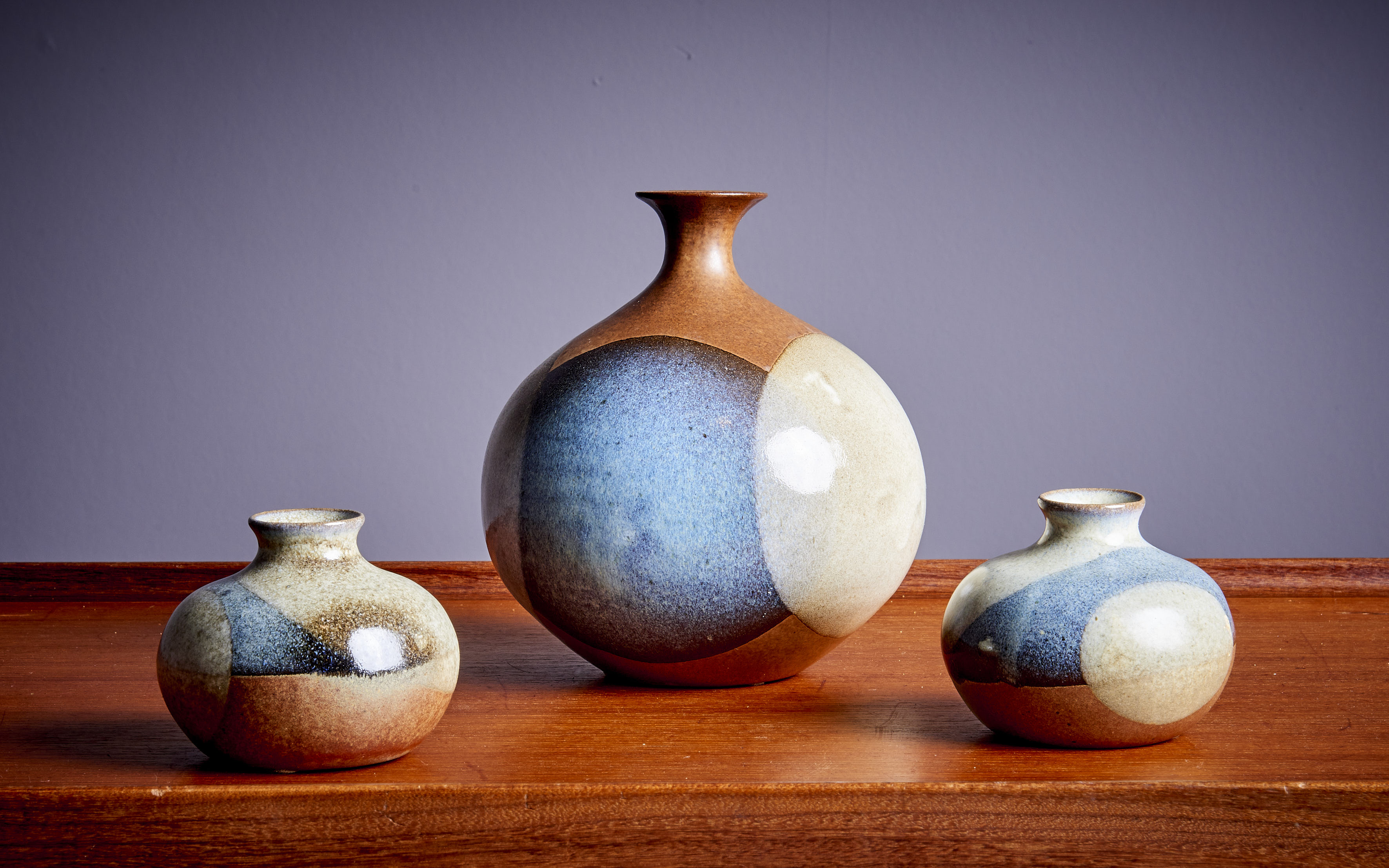This image features three distinctly patterned pottery vases arranged on a wooden table against a light purple background. The two smaller vases, positioned on the left and right, exhibit a combination of geometric shapes in shades of gray, blue, and brown, with the vase on the left showcasing slightly more blue and the vase on the right exhibiting more tan hues. Both small vases are considerably smaller, approximately half the size of the prominent large vase in the center. The central vase is striking with its large, interlocking circular designs in blue, tan, and white, spanning much of its surface. All three vases share a smooth, glossy finish, indicating a similar glazing method. The vases feature narrow openings at the top and more bulbous, rounded bottoms, creating a cohesive yet individually unique visual presentation. The entire setup is brightly lit, causing reflections on the vases' surfaces, adding to their overall appeal.